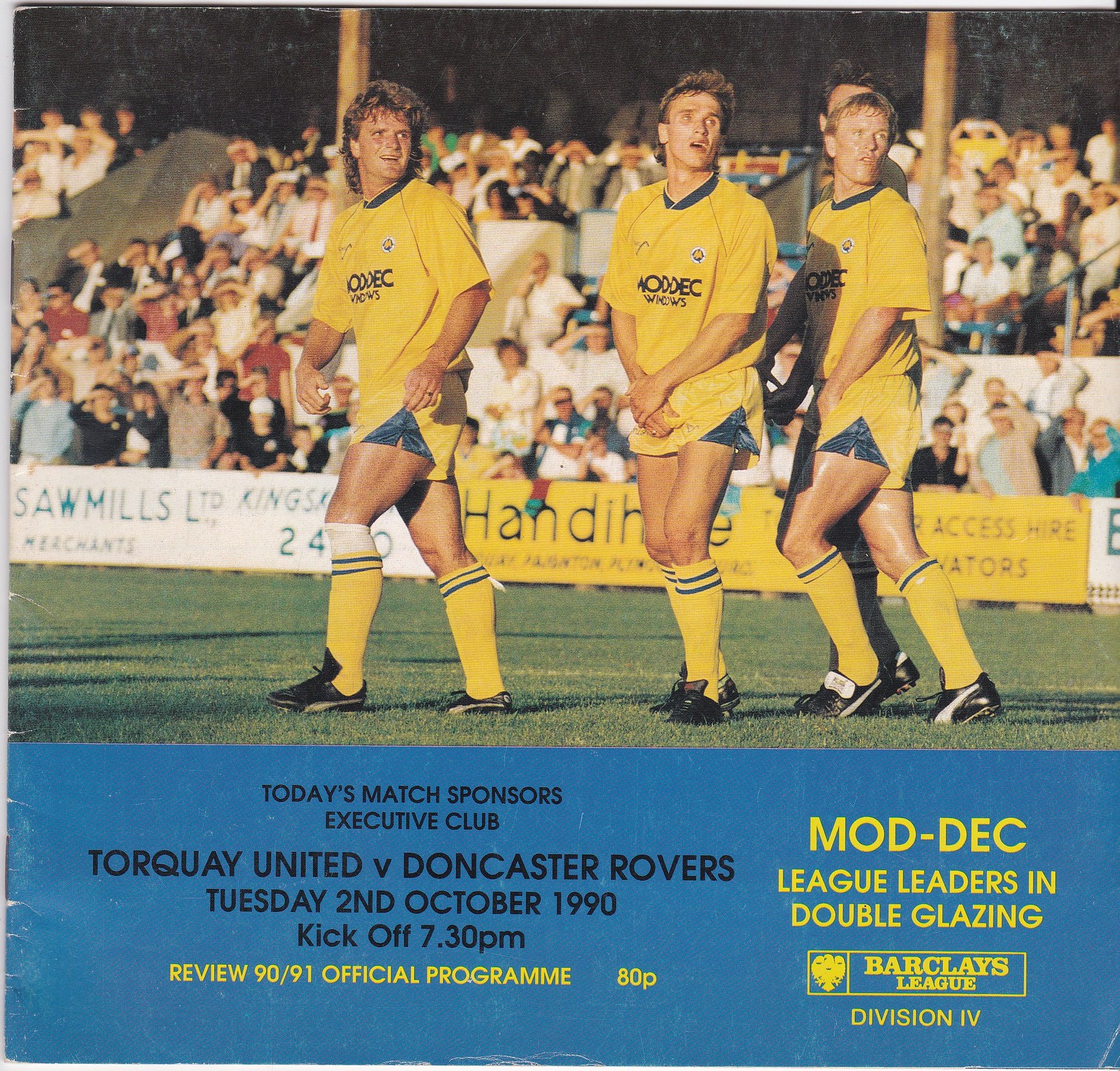The image is a detailed page from an official program for a soccer game, prominently featuring three young soccer players standing on a soccer field. The athletes are attired in yellow shirts, blue shorts, yellow socks, and dark shoes with some having white stripes. Their attention is directed towards a grandstand packed with spectators, many of whom are shielding their eyes from the bright sun with their hands. Along the bottom of the grandstand, banners display various advertisements, with backgrounds alternating between yellow and white.

The bottom section of the page includes a blue horizontal bar with text detailing the fixture: "Today's match sponsors Executive Club Torquay United vs. Doncaster Rovers," indicating the match is set for Tuesday, October 2nd, 1990, with a 7:30 PM kickoff. The text highlights the program title "Review 90/91 Official Program ADP" in yellow letters. Additionally, there's an advertisement noting the league leaders in double glazing, featuring Mark Dick.